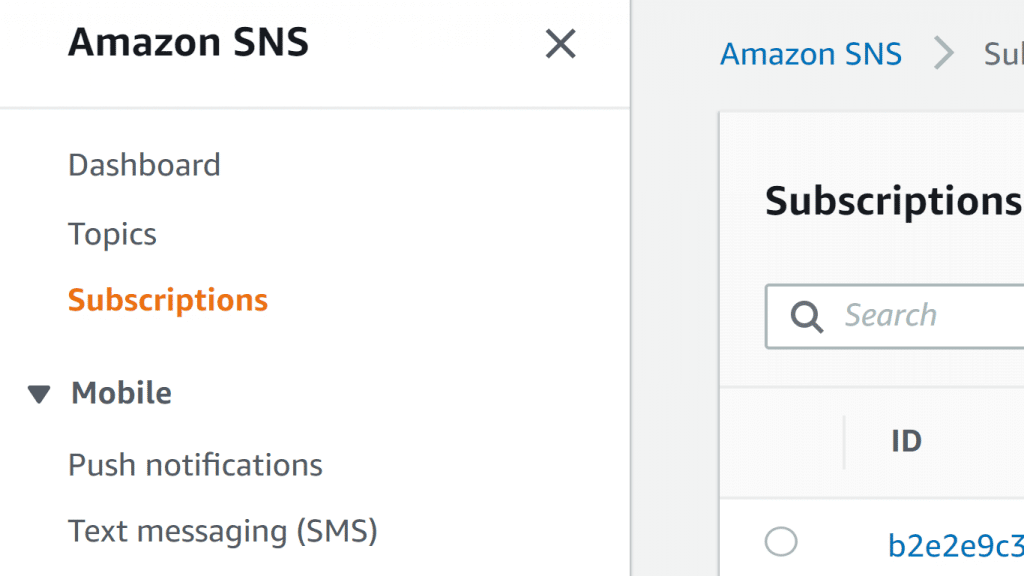The image appears to be a screenshot captured from a digital device such as a cell phone, tablet, or computer. The screenshot specifically focuses on the Amazon SNS (Simple Notification Service) interface. At the top of the screen, "Amazon SNS" is displayed, accompanied by a small 'X' in the upper right corner, likely for closing the window. Below this, a faint gray line separates the top section from the rest of the interface. 

As we move down, the menu options "Dashboard," "Topics," and "Subscriptions" are listed vertically. Notably, the word "Subscriptions" is highlighted in red, whereas "Dashboard" and "Topics" are in dark gray. Further down, there is a black arrow pointing downward next to the word "Mobile." This is followed by "Push Notifications" and "Text Messaging," with "SMS" in parentheses.

To the right part of the screen, another panel appears to be open. The top of this panel also features the title "Amazon SNS" but in blue text. An arrow points towards a partially visible word starting with "SU," which likely stands for "Subscriptions," though the text is cut off. Below this, there is a section titled "Subscriptions" in black text, accompanied by a search bar. Additionally, there is a label "ID" followed by a blue alphanumeric code reading "B2E2E9C3."